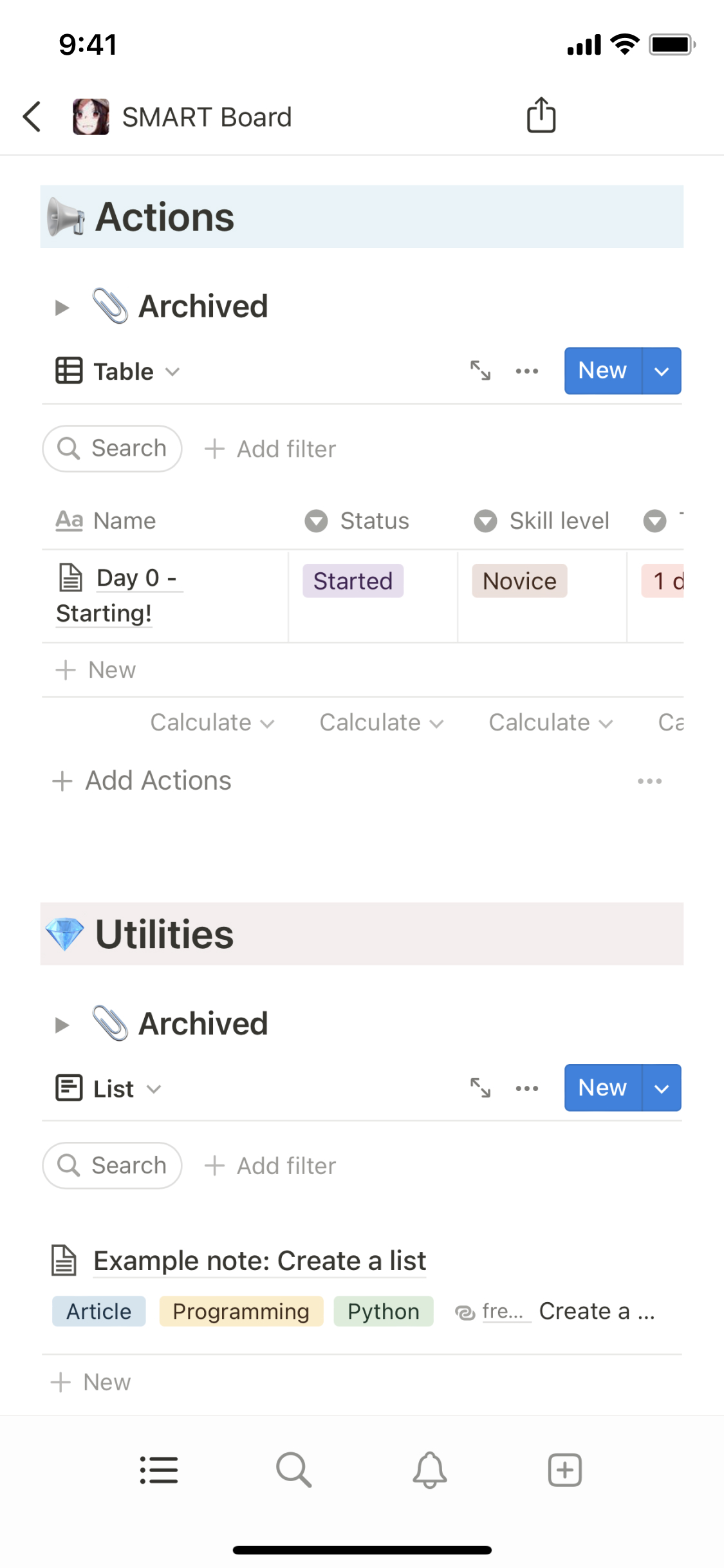The image is a detailed screenshot of a smartphone screen displaying an application interface. The app is identified as "Smart Board," with "SMART" in all caps and "Board" with an initial capital letter, located at the top left of the screen. The time displayed on the screen is 9:41, and the battery icon at the top right shows a full charge.

Below the "Smart Board" header, there are options such as "Actions" and "Archived." The interface features a tab labeled "Table," and includes a search bar accompanied by an "Add Filter" button, marked by a plus sign. 

The screen shows a table or list starting with "Day Zero," which has the following attributes:
- Status: Started
- Skill Level: Novice

Due to the layout of the screenshot, additional sections to the right are partially obscured.

There is a prominently placed "+ New" button, likely for adding new entries or categories. Furthermore, there is an "Add Actions" button, alongside multiple "Calculate" buttons, one for each column.

Below the table, there is a "Utilities" section featuring an "Archived" option and the capability to create another list based on utilities.